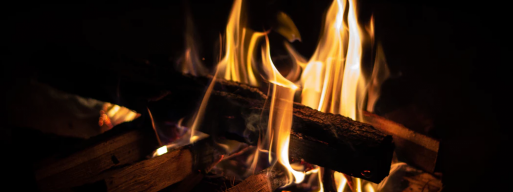The image depicts a vibrant campfire set against the jet black backdrop of night. At the heart of the fire are crisscrossed logs, forming a tic-tac-toe-like pattern, with at least three logs on each side. Flames, ranging from bright yellow to deep orange and red, energetically lick and dance around the wood. One large, half-burnt log stands out, positioned diagonally from the bottom left up towards the right corner, with flames enveloping it and shooting upwards. Warm embers glow beneath the logs, feeding the fire. The scene, viewed from a crosswise perspective at fire level, lacks any visible fire pit edges, adding to its rustic and serene outdoor ambiance.